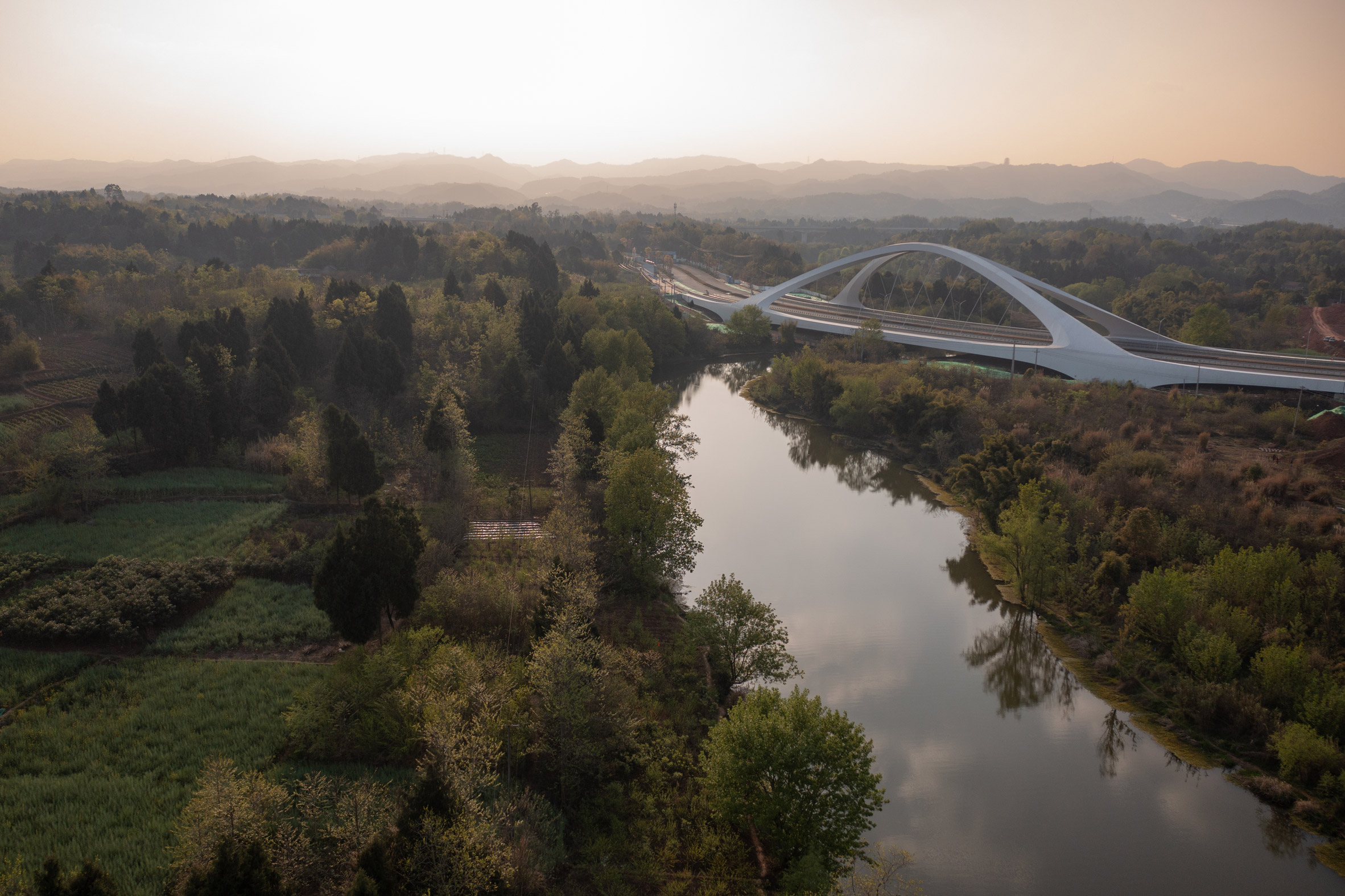This aerial photograph captures a picturesque landscape at dusk, with a gentle glow of the setting sun casting a soft light over the scene. The central feature is a river that meanders from the bottom right of the image towards the middle, its surface reflecting a mix of clouds and surrounding trees, giving it a somewhat white appearance with reflective patches. On the left side of the river, the land is adorned with a variety of greenery, including fields with low-lying vegetation and large trees, transitioning into rolling hills towards the horizon. On the right side, a striking modern bridge spans the river, curving gracefully into the sky with two prominent arching structures that almost touch at their peaks. This bridge, designed for cars or possibly a high-speed tram, adds a contemporary touch to the otherwise natural scene. The sky above transitions from pale pink on the left and right sides to a brighter area in the center, enhancing the serene, evening atmosphere of this luscious green landscape.